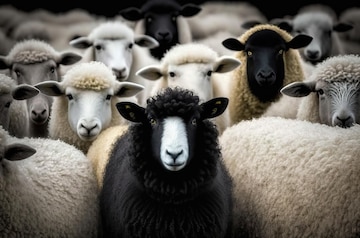A closely packed group of sheep fills the image, standing shoulder to shoulder, all intently staring at the camera. Most of the sheep feature wool coats that are predominantly white, off-white, or light beige with a yellowish tint, although a couple of sheep have black faces contrasting with their lighter wool. One particular sheep stands out in the center: a black sheep with a distinct white muzzle and striking brown eyes. Its ears are perked up, focusing directly toward the viewer, mirroring the attentive stance of the surrounding herd. The backdrop is filled with more sheep, but they appear slightly blurred, enhancing the focus on the central black sheep and its immediate neighbors. This close-knit assembly of varying hues and facial markings provides a captivating tableau of woolly, watchful faces.